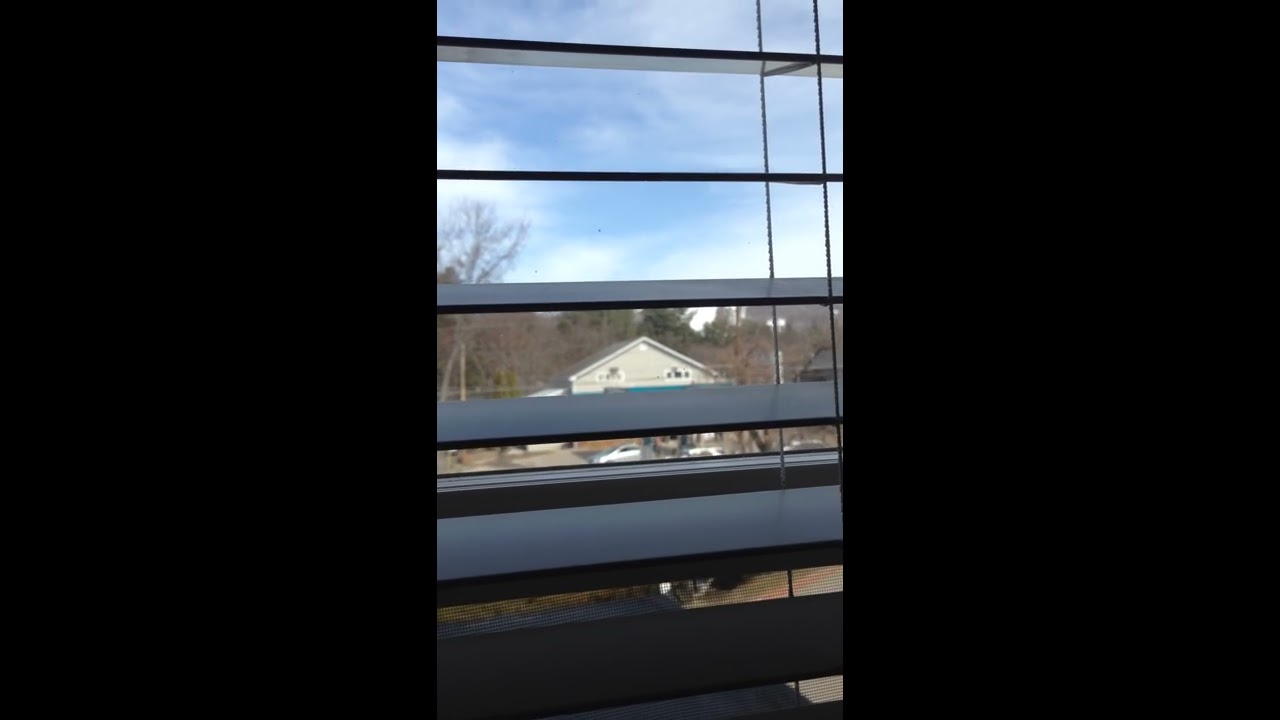This image captures a detailed view through a window from an indoor perspective, oriented vertically in portrait mode and bordered by two black bars on either side. The window's blinds are mostly down but open enough to reveal an outside scene, with the pull string on the right side. The upper half of the image highlights a partly cloudy blue sky, while the lower half displays the roofline of a beige house with a gray, triangular roof that features an attic window. Below, a silver or light blue coupe sedan is parked in front of the home’s driveway. To the left center, a deciduous tree, bare of leaves, stretches its branches towards the sky. Additional details include white planks on the house’s exterior and a background of foliage, with some trees either fully bare or having brown leaves, suggesting an autumn setting. The entire scene is framed symmetrically, offering a balanced view of suburban tranquility through the slightly tilted horizontal blinds.